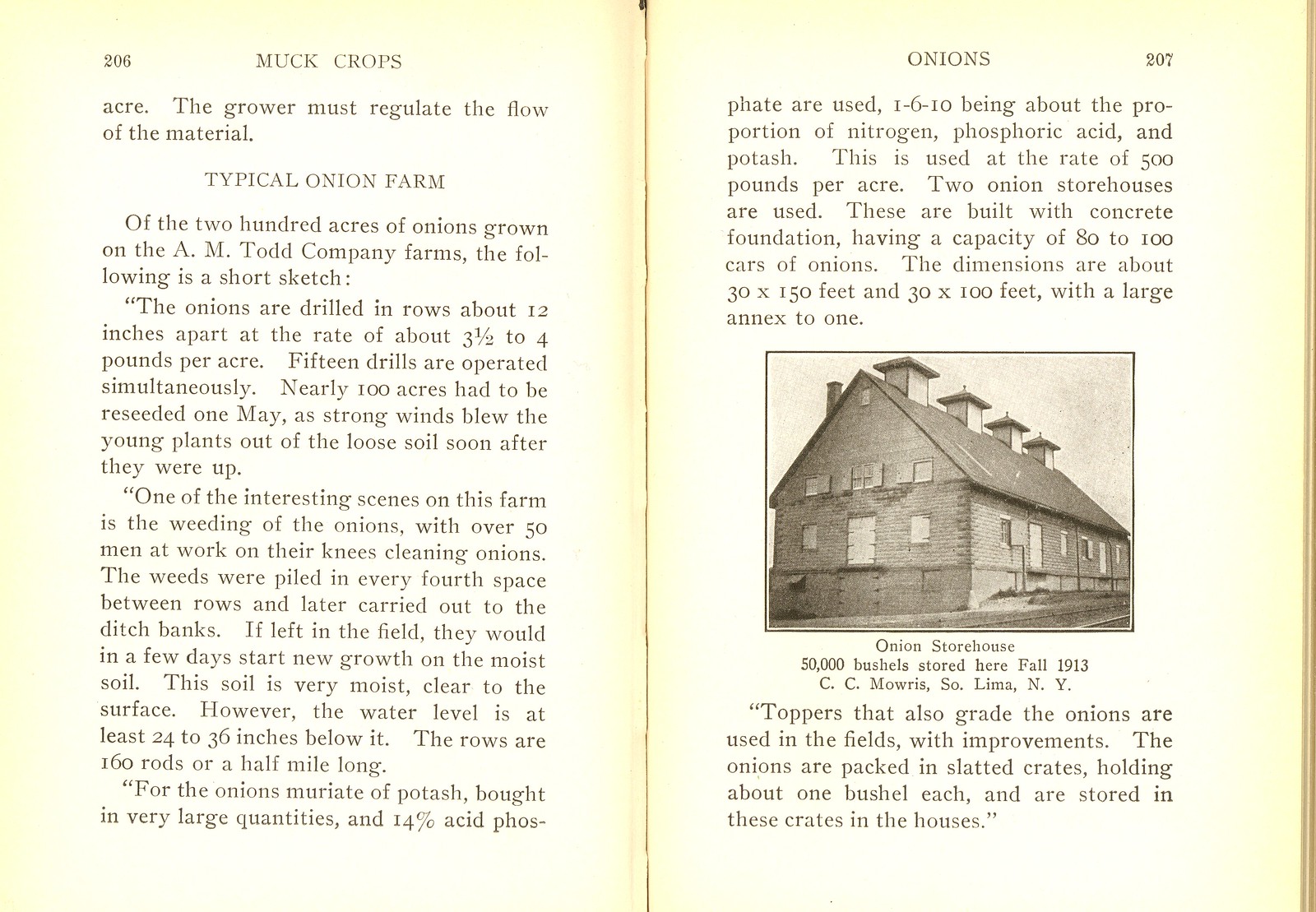The photograph captures an opened, yellowed book displaying page 206 on the left and page 207 on the right. The left page, titled "Muck Crops," contains a subsection "Acre," stating "The grower must regulate the flow of minerals." Below this, it starts with "Typical Onion Farm" and describes, "After 200 acres of onions grown on the A.M. Todd Company Farms, the following is a short sketch." The right page, numbered 207, is headed with "Onions" and features a black-and-white image of a two-story building identified as an onion storehouse. The building has four chimneys on the front and a smaller one at the back, captioned, "Onion storehouse, 50,000 bushels stored here, fall 1913, C.C. Morris, S.O., Lima, New York." The spread, characterized by its timeworn, yellowed edges, indicates an old book, likely detailing historical aspects of onion farming.